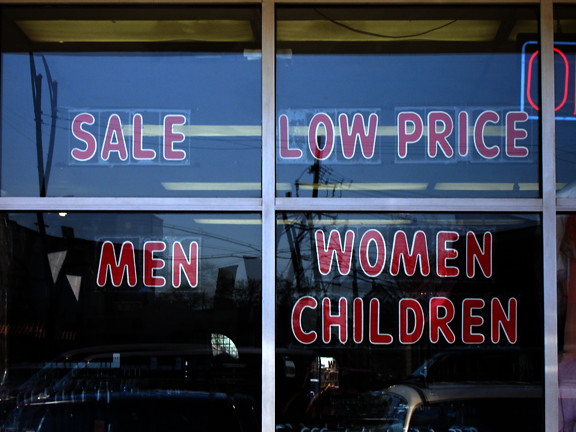The image depicts the exterior of a storefront captured in a close-up view featuring large pane windows separated by vertical and horizontal silver beams. The storefront has four window panels arranged in a 2x2 grid. In the upper left panel, bold red letters with a white outline spell out "SALE." The adjacent upper right panel similarly displays "LOW PRICE." Moving to the bottom panels, the lower left reads "MEN," while the lower right reads "WOMEN, CHILDREN," all in the same red and white sticker format. In the upper right corner, a partial 'O' in red, outlined with blue, suggests the presence of an 'OPEN' sign. The windows also capture reflections of power lines and the store's interior ceiling, revealing rectangular yellow lights. An orange, oval-shaped fluorescent light is visible on the other side of the glass, adding to the illuminated detail from within.